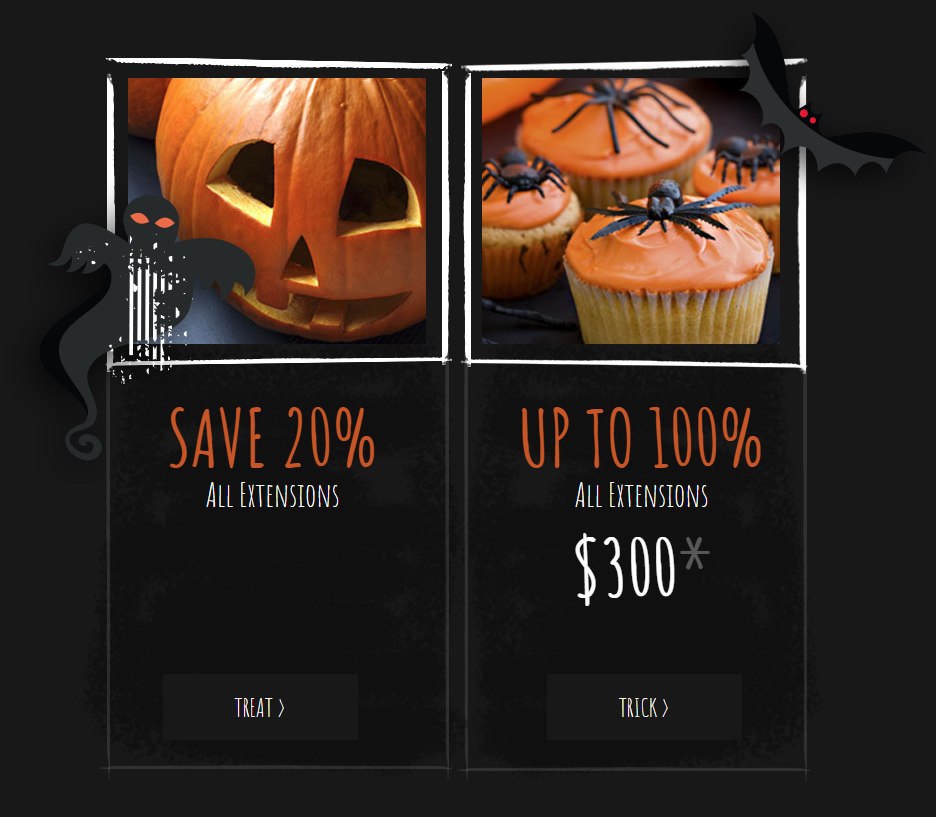The Halloween-themed advertisement features a festive layout with distinct imagery and promotional details. On the left side, a carved pumpkin is prominently displayed above a text offering "Save 20% on all extensions." Beneath this, a button labeled "Treat" invites further interaction. On the right side, a trio of vanilla cupcakes topped with orange frosting and cute spider decorations are showcased. Below this image, the text advertises "Up to 100% on all extensions" along with a price of "$300" accompanied by a small asterisk. A button labeled "Trick" is situated at the bottom. Adding to the spooky theme, a bat with piercing red eyes hovers in the upper right corner, while a black ghost with glowing orange eyes and intersecting white lines adds an eerie touch near the left side of the advertisement.